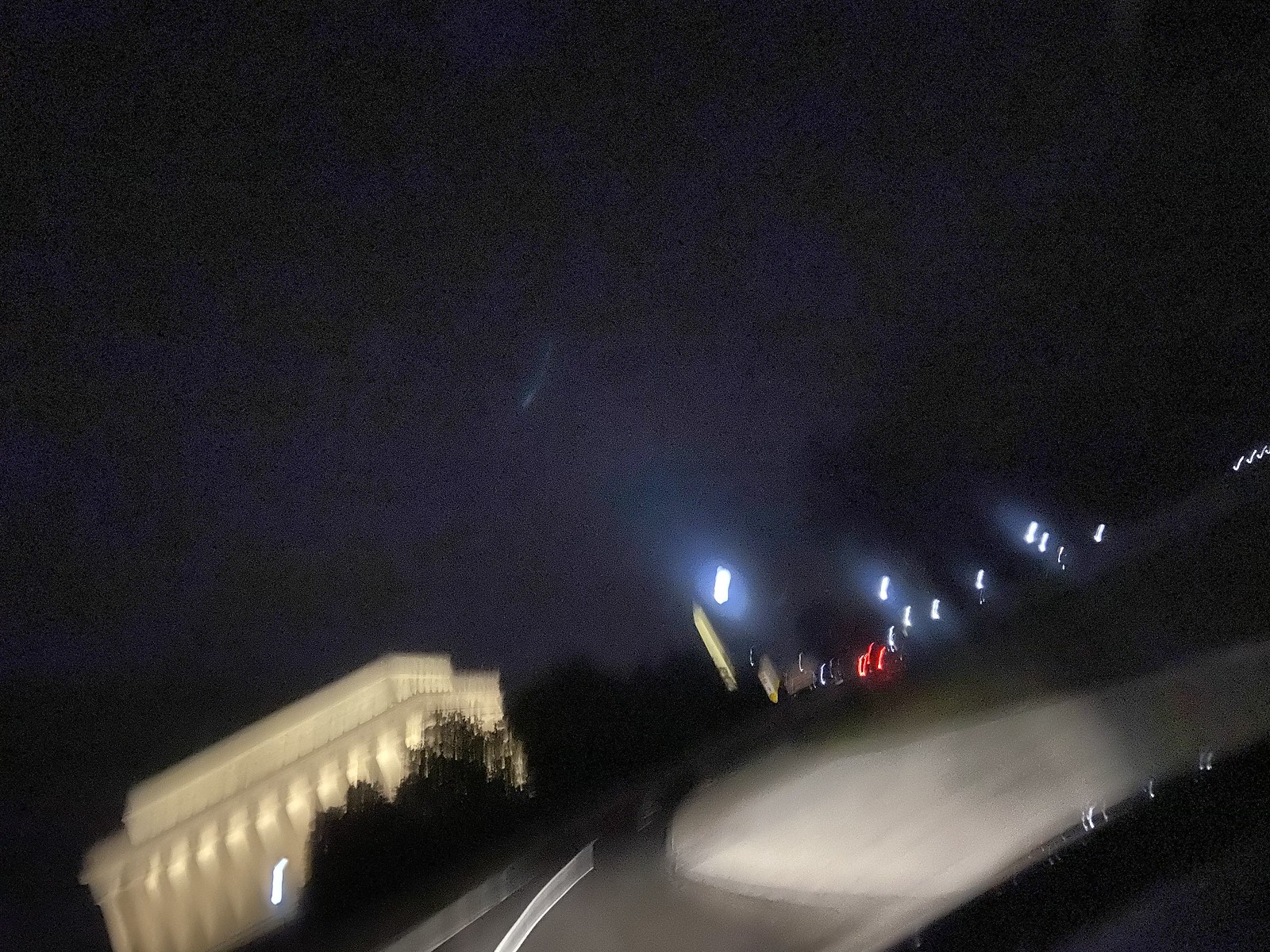This nighttime photograph, taken from a moving car in Washington, D.C., is blurry and dimly lit. The image captures a scene through the windshield with the road ahead and a white line down the middle. To the left, a well-lit, white building with many columns dominates, resembling a government structure, possibly the back of the Lincoln Memorial. A conspicuous large white spire in the background hints at the Washington Monument. The right side features scattered lights in white, red, and blue, emerging as vague rectangular shapes against the dark night. The scene is devoid of people and other vehicles, suggesting it may be taken late at night, possibly on a quiet weekend. The overall photograph has a tilt and showcases the ambient glow of streetlights, adding to the blurry, motion-captured aesthetic.